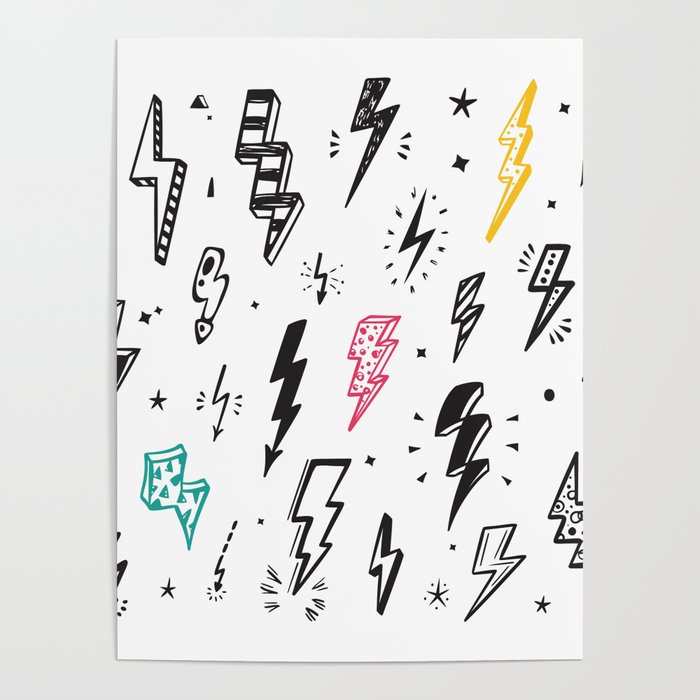This image features a white sheet of paper set against a gray background, filled with approximately 15 diverse lightning bolt drawings. The lightning bolts vary in style and color, with most being black and white. The designs include solid black bolts, black-and-white striped patterns, polka dots, and diagonal stripes. Three bolts are colored: a yellow one at the top right, a pink one in the center, and a teal one at the bottom left. The lightning bolts predominantly follow a downward zigzag trajectory from top right to bottom left. Additional details include various shapes, like some bolts looking like Swiss cheese or a pizza slice. The image also contains simple star drawings—both four-pointed and five-pointed—scattered among the lightning bolts, adding to the eclectic mix of designs. There is no text in the image.